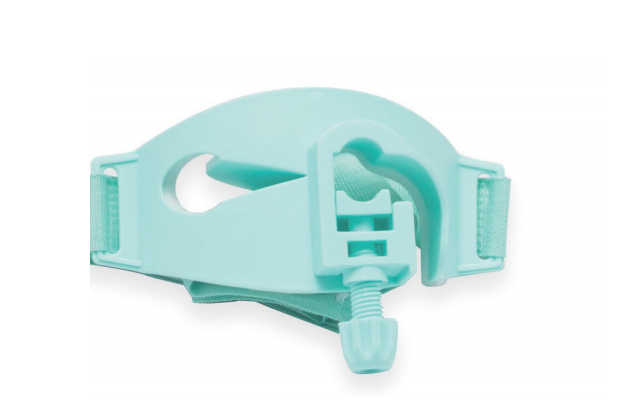The image depicts a light blue or teal-colored object, possibly made of silicone or a similar soft material, placed against a white background. The object resembles a vise or a belt buckle with a screw mechanism at its lower middle portion. This screw, which appears to be plastic, protrudes vertically and facilitates a clamping function. The object is approximately 8 inches in size, with a rounded top and two slits on either side that allow a strap or fabric to pass through. The overall impression is of a versatile, clamp-like contraption with a smooth, soft texture and a curved design.